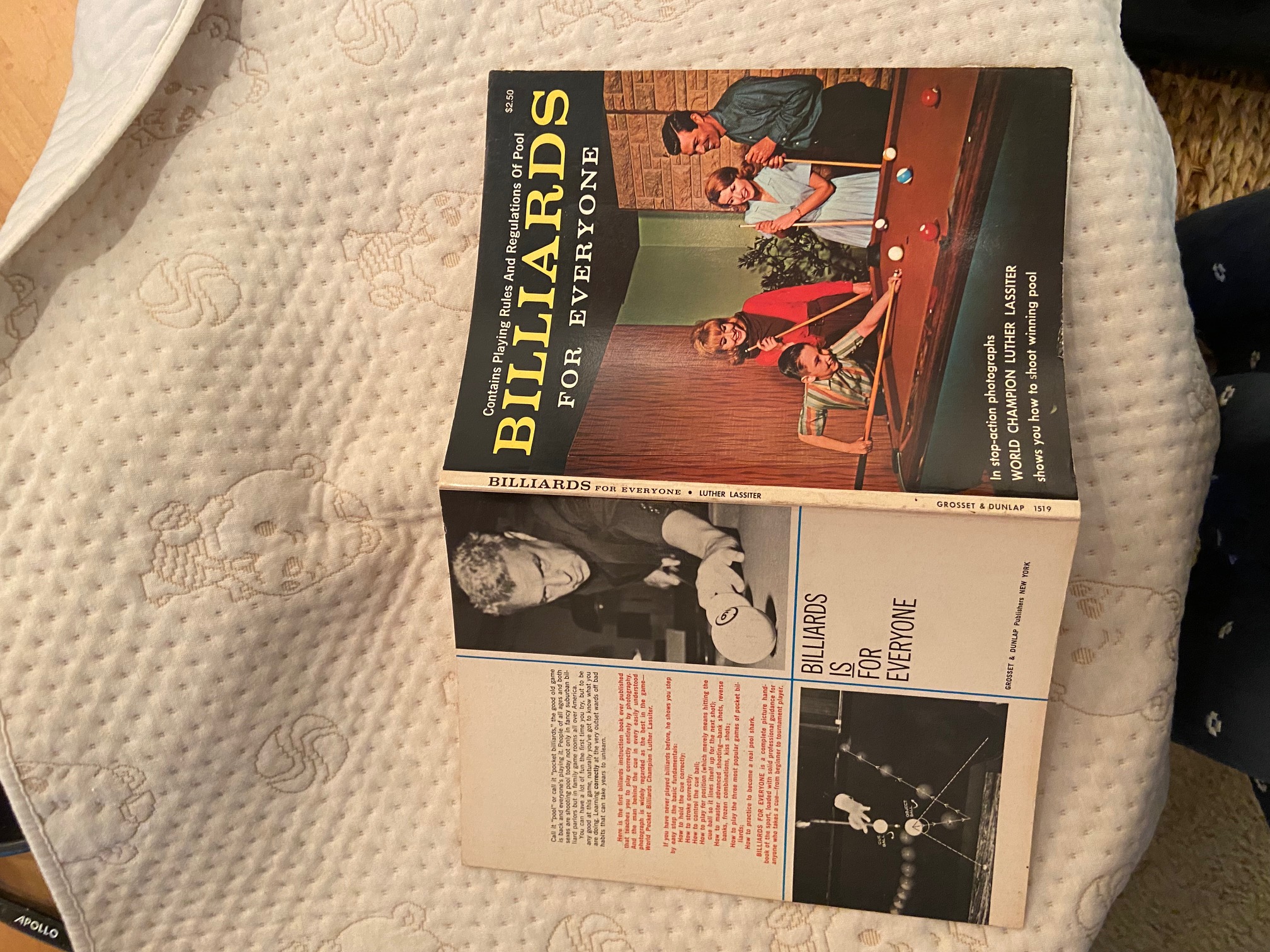The image depicts a book titled "Billiards for Everyone," which is open and lying face down on a white cloth decorated with small designs such as teddy bears and balls. The cover of the book features a colorful picture of a family playing pool, including a man, a woman in a dress with blonde hair and a red shirt, and a child. The book's title is prominently displayed in yellow and white letters, with additional text indicating that it contains the playing rules and regulations of pool and is priced at $2.50. The top of the book also mentions "In Step Action Photographs World Champion Luther Lassiter shows you how to shoot winning pool." The background of the image includes a small piece of wood in the top left corner and something dark on the right. On the back cover of the book, there are black and white photographs.